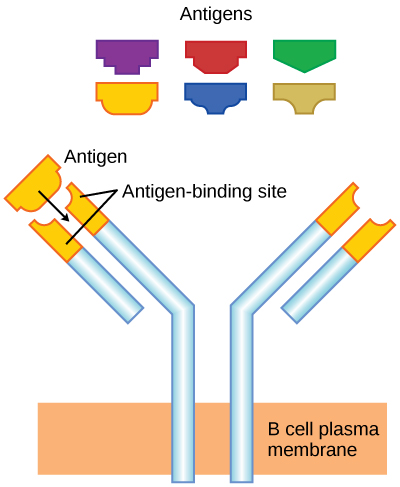The diagram is a detailed medical graphic illustrating antigen binding to an antigen-binding site. At the top, labeled "antigens," are six distinct polygons of different colors: red, purple, green, yellow, blue, and tan, each with unique edge shapes. These antigens funnel through a white, L-shaped pipe that represents the B-cell plasma membrane. The membrane is labeled in black text on a peach-colored strip. The diagram focuses on a yellow antigen plugging into the antigen-binding site, depicted at the end of the bent pipe. Arrows indicate the binding process, showcasing how antigens interact with the B-cell plasma membrane.